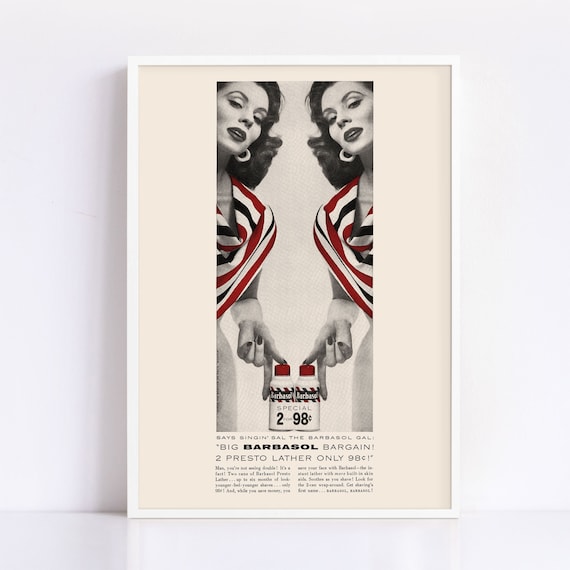This is a vintage Barbasol shaving cream advertisement, elegantly framed in white and set against a pristine white background on a white shelf. The ad itself features a cream-colored backdrop with predominantly black and white imagery, accented with strategic splashes of red. Central to the ad are two identical images of the same heavily made-up woman, adorned with large hoop earrings and curling long brown hair, giving the impression of a mirror image. Each woman has a poised finger resting on one of the two red-capped Barbasol cans, which prominently display the text "special, two for 98 cents" and "big Barbasol bargain, two Presto lather only 98 cents." Their flowing blouses expertly mix white, black, and red stripes, echoing the red stripes on the Barbasol labels. The only colors in the ad are the vivid red highlights in the woman's blouse and the Barbasol cans, creating a striking contrast against the mostly monochromatic scheme. Additional smaller text appears in two columns, though it remains too small to read.